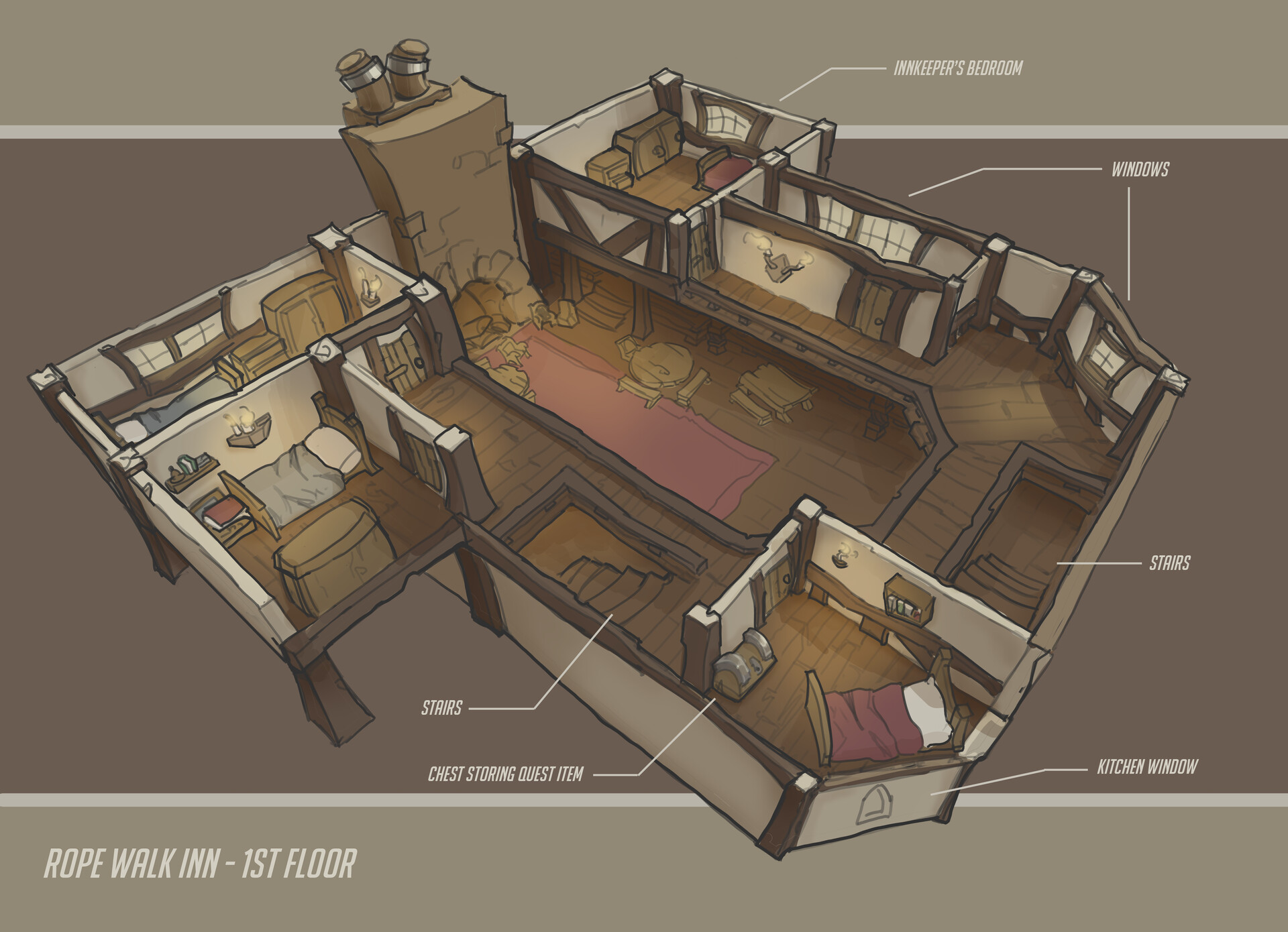This image is a detailed aerial diagram of a house, rendered as though from a video game. The diagram spans two floors, focusing here on the first floor labeled as "Rope Walk-In - First Floor" in white text on a gray section at the bottom. The house features multiple bedrooms, each equipped with beds of varying sizes and colors such as blue, gray, and possibly purple, all with white pillows. The rooms also include brown wooden dressers. The walls are depicted in white, with brown wooden flooring and stairs.

In the central area, there's a fireplace made of tan or brownish stones or bricks. The fireplace is surrounded by an open balcony-like structure. The house includes windows strategically placed around the diagram, emphasizing its residential nature.

The detailed labels on the floor plan identify specific areas: the innkeeper's bedroom at the top, a kitchen window, and multiple stairs indicating a second floor. There is also a chest labeled for storing quest items. Additional features include brown wooden tables and chairs, and a red carpet on the floor. The visual elements and labeling hint at an inn-like setting, possibly within a video game environment.